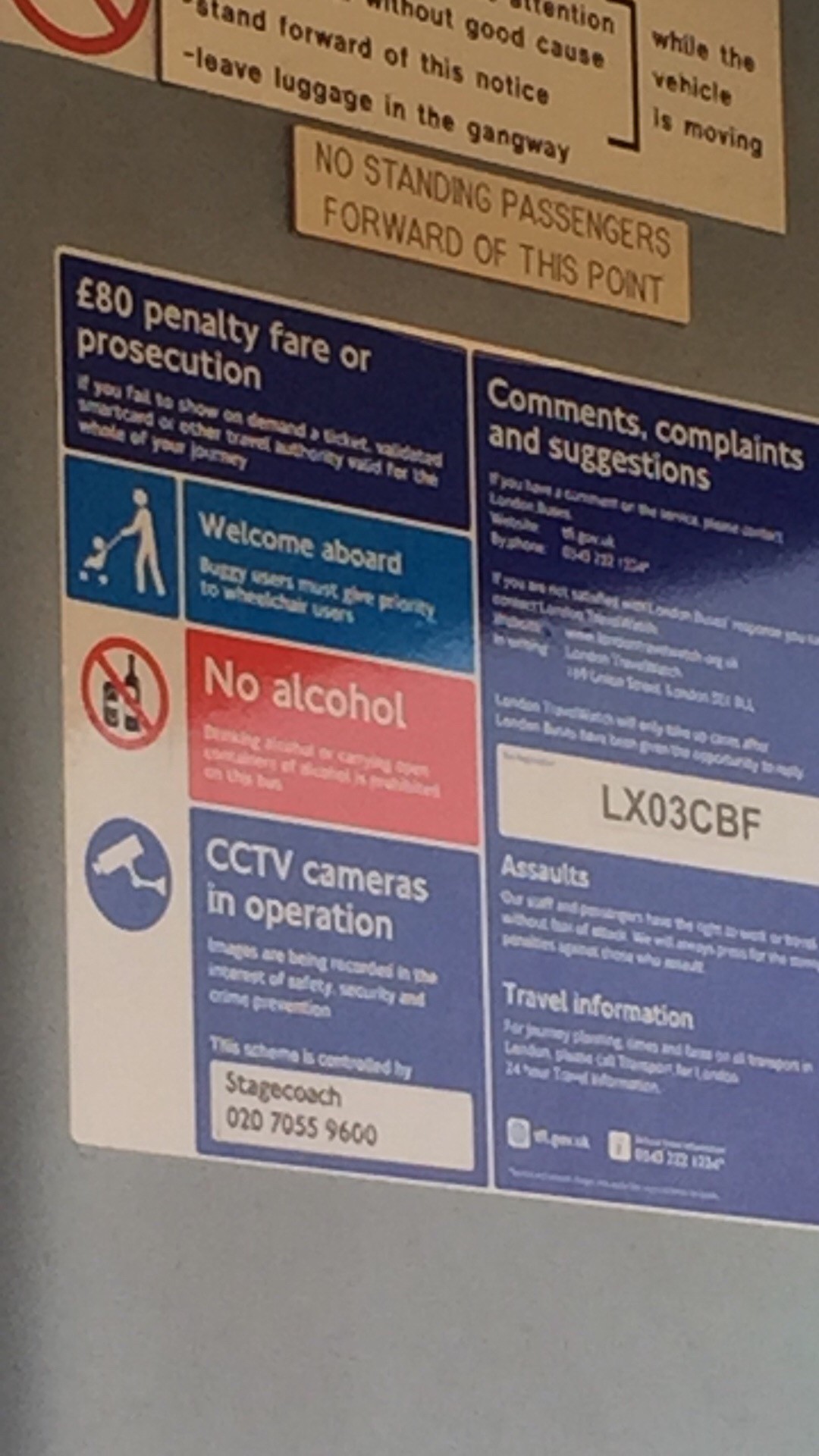The image depicts a series of informational signs affixed to a grey wall, likely located in a public transportation setting such as an airport. At the top, there's a white sign partially visible with text including "Leave luggage in the gangway." Below it, a smaller white or off-white sign reads, "No standing passengers forward of this point." The largest and most detailed sign, blue in color, features multiple sections. The top section warns of an "80 pound penalty, fare or prosecution" with implications for certain infractions. The middle sections include a welcoming message, "Welcome aboard," and an image of an adult pushing a child in a stroller. Following that, a red section explicitly prohibits alcohol, depicted by a crossed-out wine bottle graphic. Further down, the sign indicates that "CCTV cameras in operation," accompanied by an icon of a camera. Additional text in the top right corner of the blue sign includes "Comments, complaints, and suggestions," and a license plate-like code, "LX03CBF," is displayed prominently in the middle section.